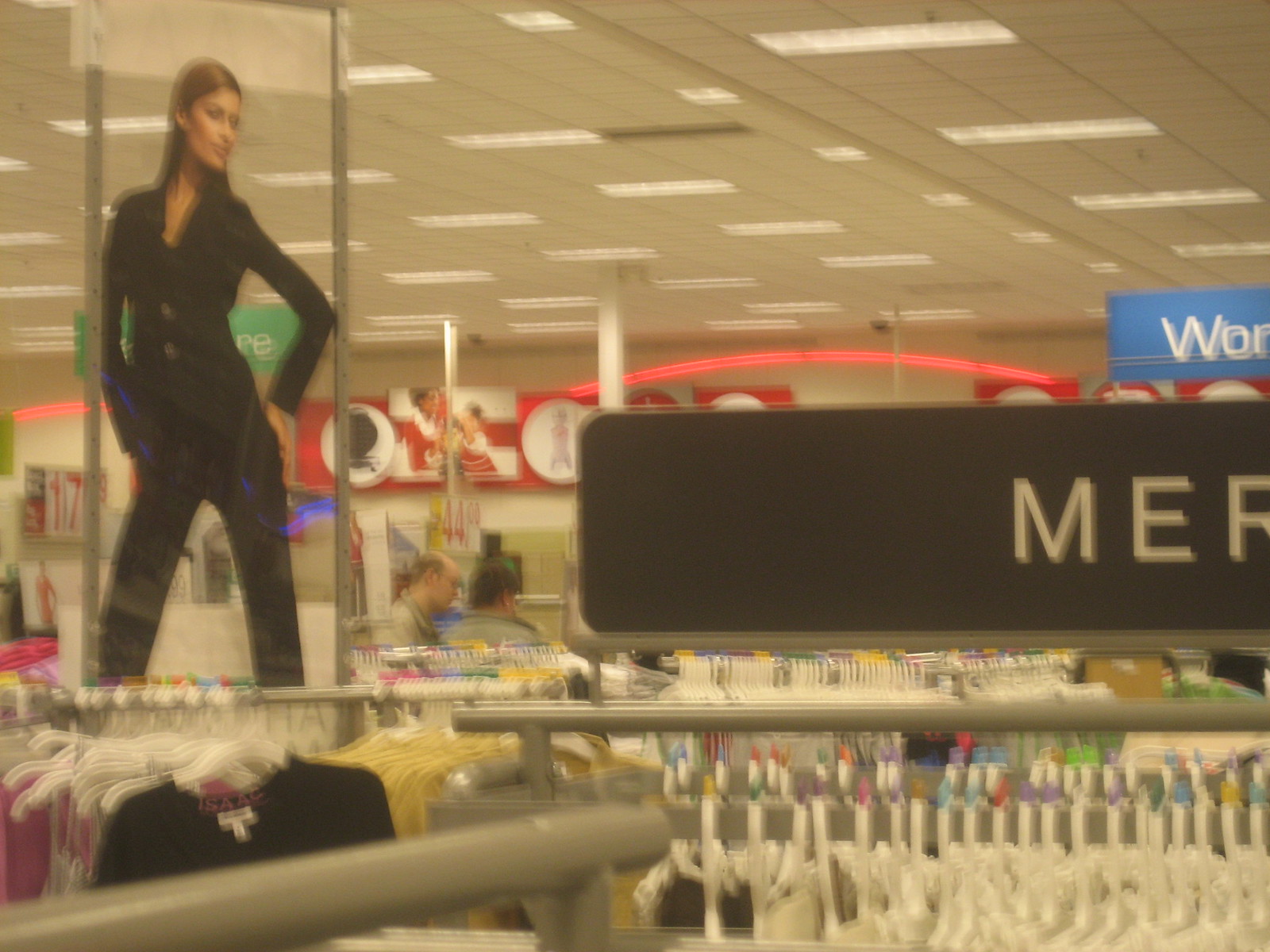This horizontal, low-resolution photograph captures the bustling interior of a retail store, likely a department store. In the foreground, chrome-colored metal racks are crowded with women's clothing items hung on white hangers, each adorned with multicolored size markers—pink, blue, red, green, and yellow. A prominent black sign with white letters reads "M-E-R," though it's cut off, hinting at the "Women's Department" while partially obscured. Another blue sign in the background also appears incomplete, displaying "W-O" followed by an "M." A striking cardboard cutout of a Caucasian woman with long brown hair stands near the racks, depicted in a black pantsuit with her hand on her hip. The store's ceiling is composed of large acoustic tiles with inset fluorescent lighting, further illuminating the scene. There are blurred figures of shoppers moving about, and red signage hanging from the white back wall, adding to the store's vibrant atmosphere. The overall setting suggests a mid-market retail environment, with various departments and model cutout figures visible in the background.